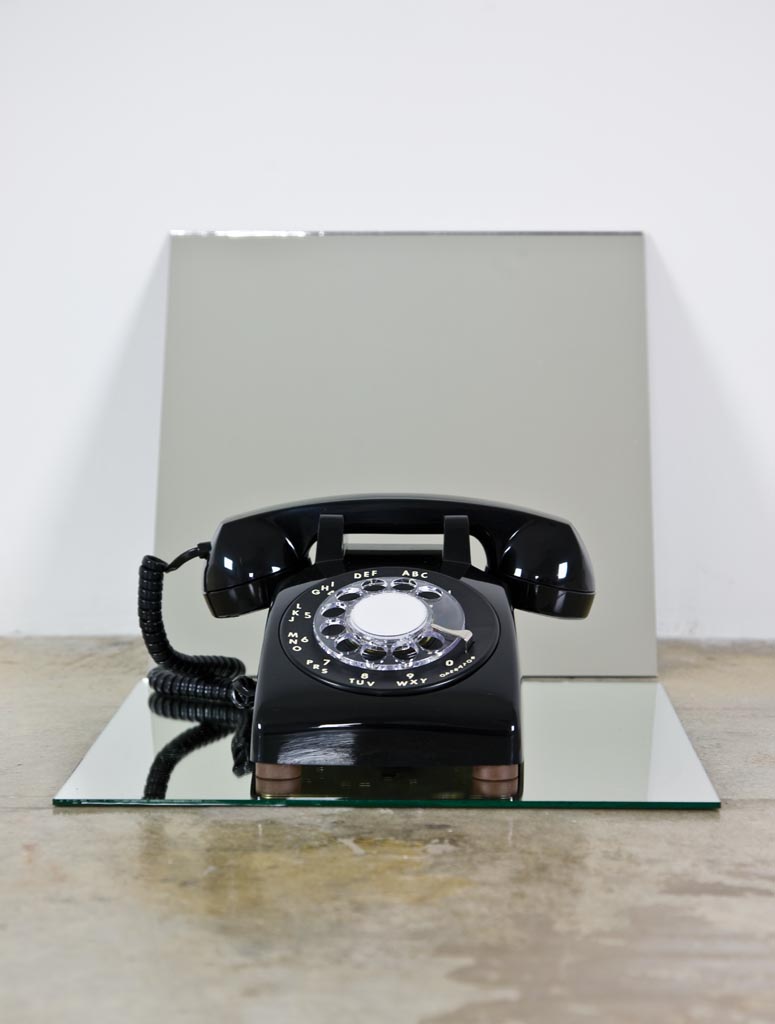The image features a shiny, black, rotary dial telephone from the 1950s-70s era, prominently displaying its white numbered dial and clear finger holes. The phone sits on a mirrored platform, reflecting parts of the phone including the cord and circular base. Behind the phone is an angled object, possibly another mirror or a grayish-white panel with a chrome stripe at the top, set against a white wall. The entire setup is situated on a brownish-gray stone surface, contributing to the vintage aesthetic.